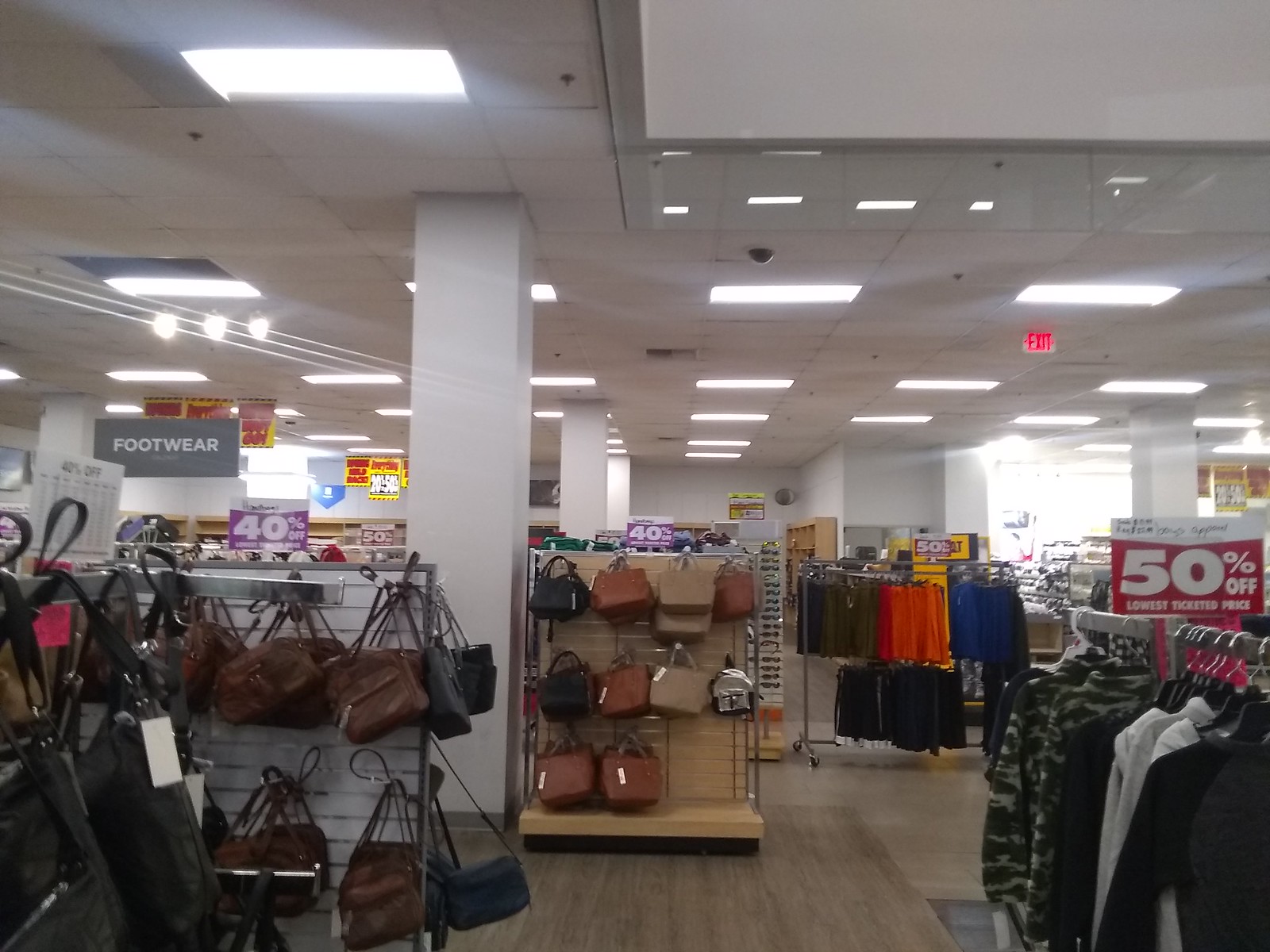This color photograph captures the interior of a large retail store with a grey ceiling featuring numerous white, squarish fluorescent lights. Prominently, there's white square beams or columns visible throughout the store, and a lit exit sign with red letters can be seen in the top right of the image. The store's layout shows a variety of displays; on the bottom left corner, there's a display of mostly brown handbags, and in the center, there's a lighter-colored wooden stand with handbags of beige, brown, and black hues. Clothing racks are scattered throughout, including athletic wear, sweaters, and jackets, with prominent red signs indicating 50% off. To the left of the center, an array of handbags and purses is displayed. In the background, footwear sections can be seen under a large grey sign labeled "footwear" in white letters. A notable detail includes a pair of bright orange basketball shorts near the front. The bottom right of the image shows a display of black and white clothing. The shop is well illuminated, and there are signs throughout, including ones indicating sales with 40% and 50% off. The flooring in the store is a light brown hardwood, adding warmth to the expansive interior.